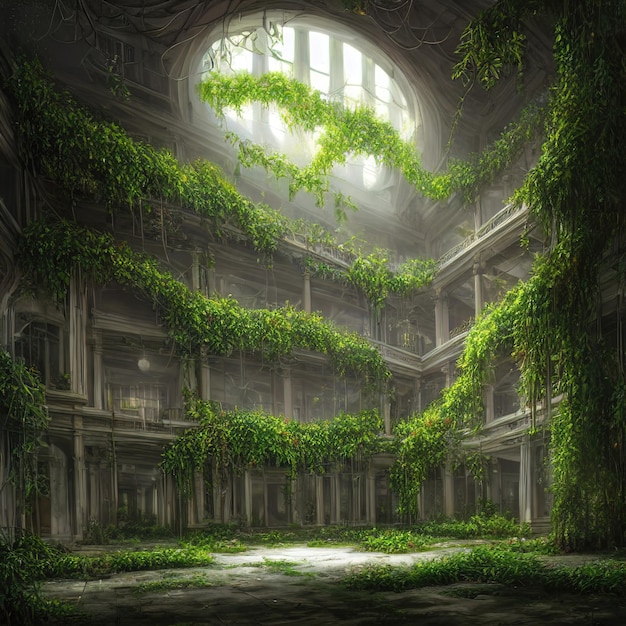The image is a detailed digital rendering of ruins overtaken by nature, resembling a post-apocalyptic scene. From an internal perspective, the scene features a large, oval-ish skylight at the top that allows bright white light to stream into the otherwise dark and decaying space. The building is multi-leveled with up to four floors, each supported by numerous vertical columns, suggesting a layout reminiscent of Japanese architecture with an open, airy design. Dense greenery, dominated by vibrant green vines, sprawls across the scene—crawling over pillars, stretching across floors, and engulfing the building completely, particularly dense on the right side. The ground below is carpeted with more greenery, emphasizing nature’s reclamation of the abandoned structure. Besides the greenery, the primary colors in the image are the dark grays of the decrepit building. On the left, a solitary lamp remains as a faint reminder of human presence in this otherwise thoroughly reclaimed environment.